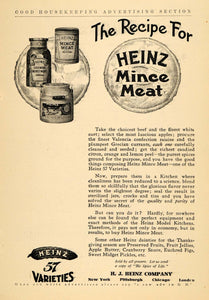This image appears to be an old advertisement, likely from the 1940s or 1950s, featuring a recipe for Heinz Mincemeat. It seems to have been clipped from a newspaper or magazine, given its yellowing paper and vintage font. At the top of the ad, "Good Housekeeping Advertising Section" is prominently displayed. The image has a pinkish background with various elements arranged on it.

In the top left corner, there are illustrations of three Heinz products—though the exact contents of the jars are unclear due to poor resolution, they are assumed to be condiments. Centered at the top is the title "The Recipe for Heinz Mincemeat," framed within a circle. Beneath this title is an illustration of a pie, with the words "Heinz Mincemeat" emblazoned across it. The actual recipe, though present, is illegible due to blurriness.

The bottom left of the ad features the classic Heinz 57 varieties logo, characterized by a black illustration of a pickle with the word "Heinz" above and "57 Varieties" below. Additionally, the signature at the bottom mentions the H.J. Heinz Company with branches in New York, Pittsburgh, and Chicago. The overall composition and aesthetic of the ad, coupled with its delicate condition, strongly suggest it is a nostalgic piece from mid-20th-century print media.